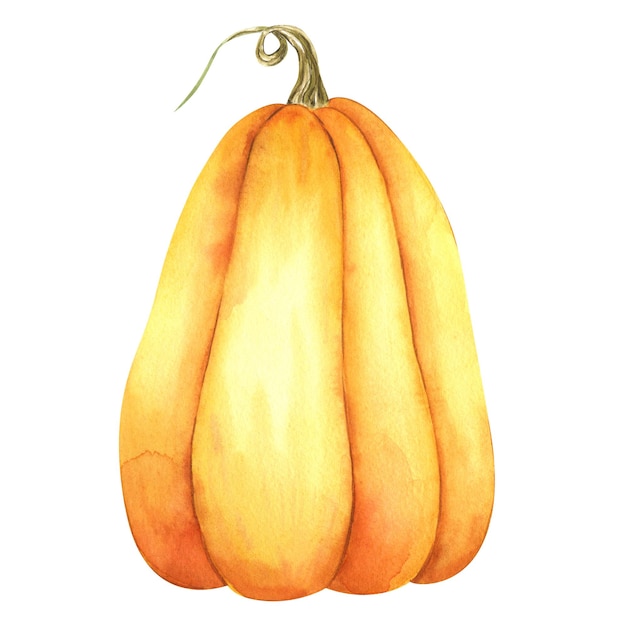This is a large colored pencil drawing of a uniquely shaped, tall and oblong gourd. The gourd is orange, featuring a gradient of colors: it starts as a darker orange at the top, transitions into a lighter orange and yellow in the middle, and darkens again towards the bottom. Three prominent ridges create four distinct sections visible from the front, adding texture and depth. The greenish stalk at the top, accentuated with white and hints of light brown, twists to the left, forming a curly Q shape before tapering into a delicate string. The gourd is set against a pristine white background that highlights its vibrant colors and intricate details.